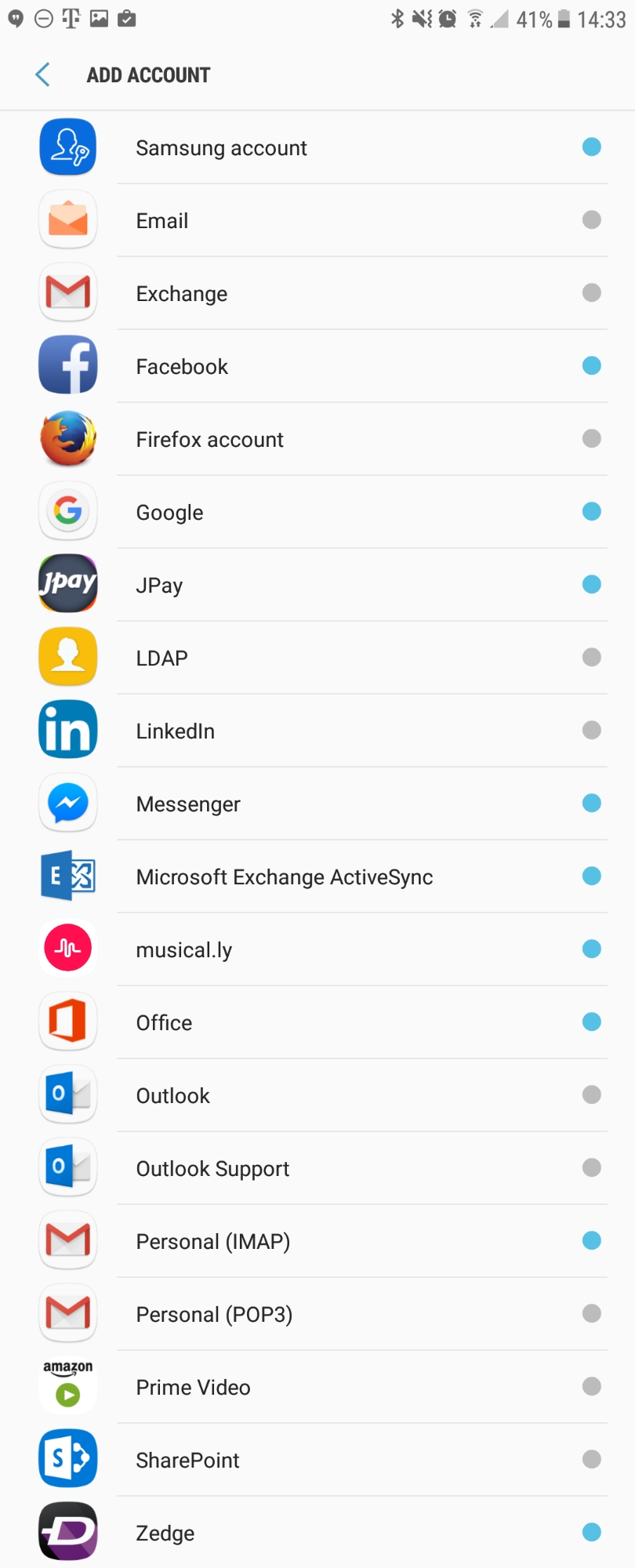This detailed screenshot from a smartphone, identified by the T-Mobile network icon in the status bar, showcases a typical account management interface. The status bar at the top features an array of icons: T-Mobile's uppercase "T" logo, a rectangular photo icon, a suitcase icon with a checkmark, Bluetooth icon, audio symbol, alarm icon, Wi-Fi signal strength, battery level at 41%, and the time indicated as 14:33. 

Below the status bar, the screen prominently displays the "Add Account" option, followed by an extensive list of account types that can be added. These accounts, listed from top to bottom, include:

1. Samsung Account
2. Email
3. Gmail (Gmail icon present)
4. Exchange
5. Facebook
6. Firefox Account
7. Google
8. J-Pay
9. LDAP (featured with a yellow icon depicting a person)
10. LinkedIn
11. Messenger
12. Microsoft Exchange ActiveSync
13. Musical.ly
14. Office
15. Outlook
16. Outlook Support
17. Gmail Personal (IMAP)
18. Gmail Personal (POP3)
19. Prime Video
20. SharePoint
21. Zedge

Each account type signifies popular platforms or services, ensuring users can seamlessly integrate various services within their smartphone's ecosystem.